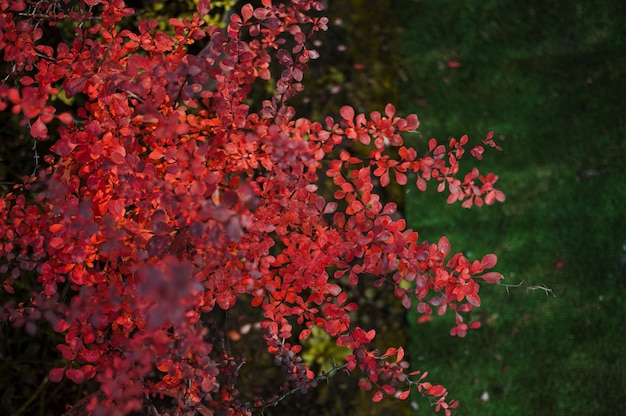This aerial photograph, likely taken by a drone about 10 feet above, captures a striking tree branch adorned with predominantly reddish leaves. The leaves exhibit shades ranging from light red to pinkish hues, intermingling with a few white leaves. The branch, occupying the left side and extending into the center of the frame, has smaller limbs that splinter off multiple times, each about two to three feet in length. Below, the neatly maintained expanse of grass, possibly indicative of a yard or city park, occupies the right side of the image. The contrast between the dark soil beneath the tree and the green grass further suggests a manicured setting. Additionally, clusters of berries are visible at the bottom of the picture, adding to the botanical details of this visually captivating scene.